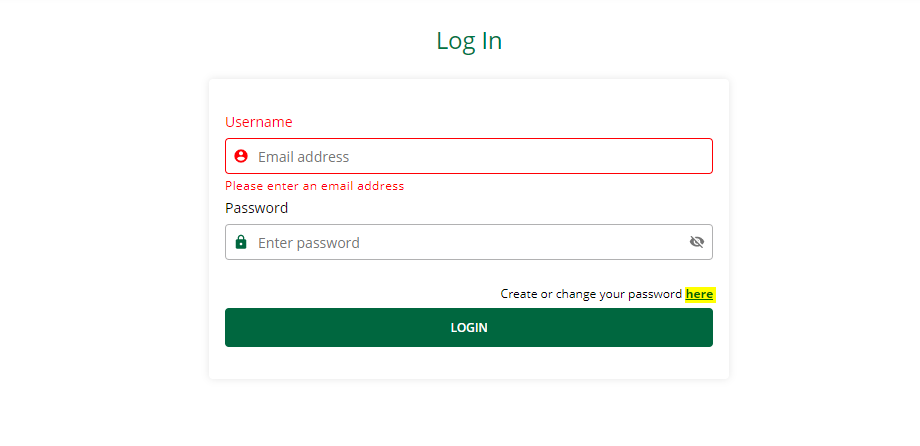A screenshot of a login interface with a clean and structured design on a white background. Centered at the top, the word "Login" is prominently displayed in large green letters. Below this, a white box outlined in light gray serves as the main container for the login fields.

Approximately three lines down from the top, the word "Username" is displayed in red on the left side, next to a red-outlined rectangle that contains a red person icon. To the right of the icon, "Email Address" is written in dark gray text. Directly beneath this, a red error message reads, "Please enter an email address."

Two lines further down, the label "Password" appears on the left in light black text. Below this label, another rectangle outlined in gray features a green lock icon on the left. To the right of the icon, lighter gray text prompts, "Enter Password." On the right end of this rectangle, there is an eye icon with a slash through it, indicating that the password is hidden.

About four or five lines below, a dark green rectangular button spans the width of the screen with "Login" centered in white text. Above this button, on the right side, small black text reads, "Create or change your password." The word "here" in this text is underlined and stands out with a potential green hue against a yellow background, indicating it as a clickable link.